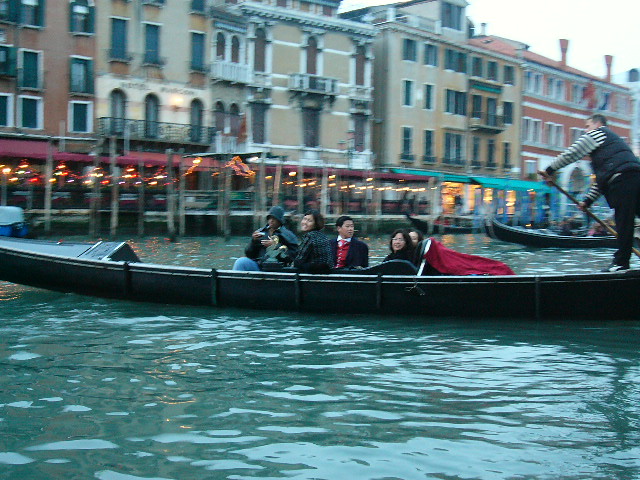In the photograph, we see a gondola gliding across a blue-green river, likely in Venice, given the presence of tightly packed, colorful buildings that line the waterway, adorned with lights and awnings from various restaurants and cafes. The gondola is a plain black or dark green vessel, steered by a gondolier in a black and white striped shirt and thick puffer vest, partially cut off from the image on the far right. There are 4 or 5 passengers, mostly Asian, sitting centrally in the gondola, appearing to enjoy their ride with smiles on their faces. In the background, slightly blurred, are additional gondolas and an array of buildings, some bustling with restaurant activity and equipped with hanging lights and tables, indicating a lively Venetian scene just as dusk begins to settle.